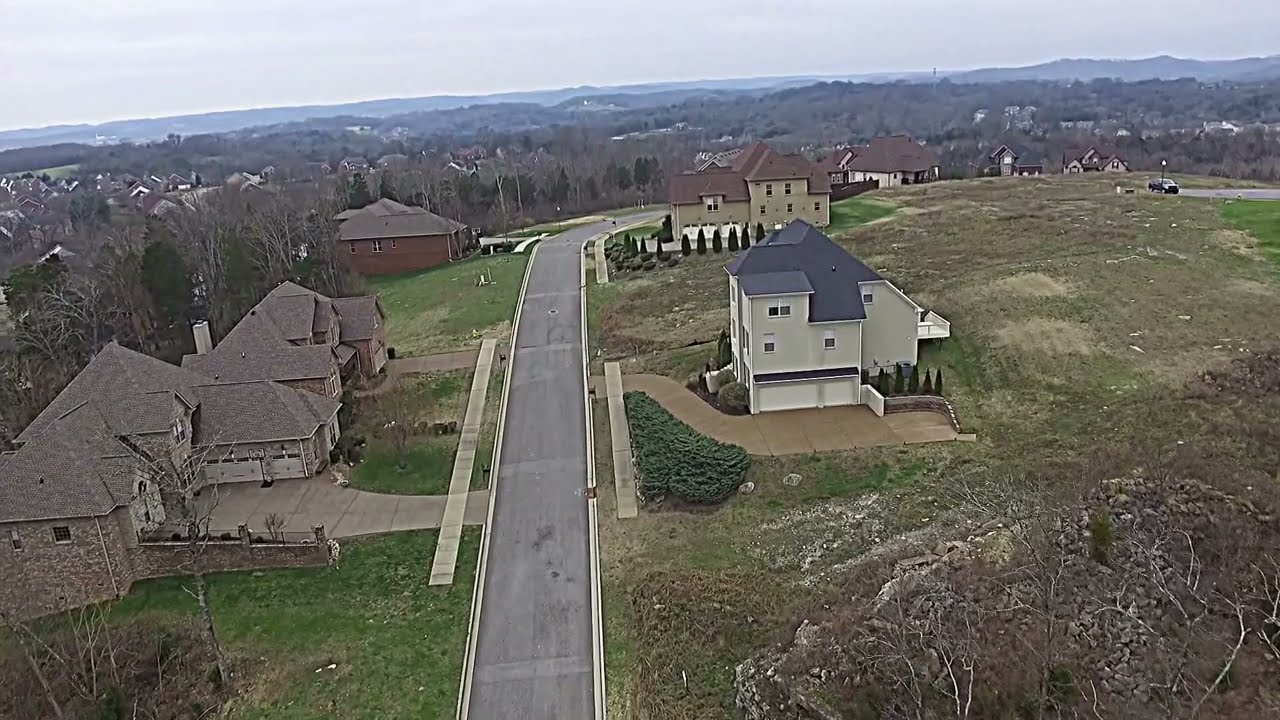The image is a landscape-oriented, color photograph taken from a drone, capturing an overhead view of a suburban neighborhood in a rural hillside setting. A prominent gray street runs down the middle, flanked by several large, two-story homes. Notably, to the bottom left, there is a very large home with a three-car garage and multiple driveways. The homes are surrounded by a mix of greenery, including grass, bushes, and trees, although the terrain shows patches of brown, muddy areas and rocky sections, particularly towards the bottom right. The background features a bluish-gray mountainscape under an overcast, grayish-blue sky, adding to the scenic, yet realistic, representational style of the photograph.